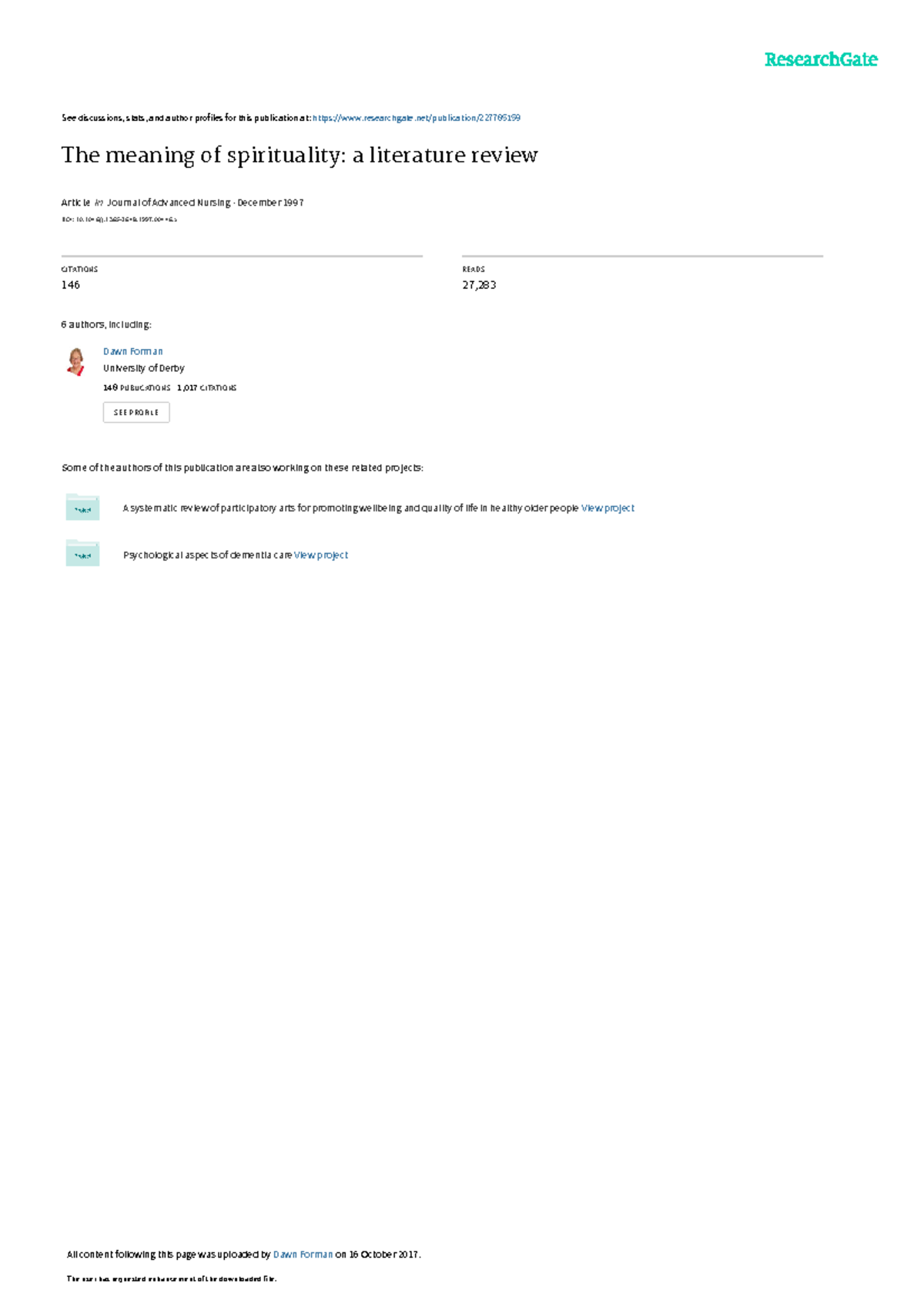The image contains a screenshot from ResearchGate, showcasing a publication titled "The Meaning of Spirituality: A Literature Review." 

In the top right corner, the name "ResearchGate" is prominently displayed, with the 'R' and 'G' capitalized and colored in turquoise. Below it, aligned to the left, there is a black text link: "See discussion stats and other profiles for this publication at https://www.researchgate.net 227785159". The hyperlink "227785159" is in blue and clickable, redirecting to the related webpage.

Further down, in large text, the title of the publication is displayed: "The Meaning of Spirituality, a Literature Review." Below the title, smaller text in bold and italics indicates the source: "Journal of Advanced Nursing December 1997," along with the article's serial numbers.

Beneath this is a horizontal line stretching from the left to the center. Below this line, the word "Citation" is mentioned with the number "146." Adjacent to this, another line stretches from the center to the right, followed by the word "Reads" and the number "27283."

Continuing down and aligned left, the text lists six authors, including a profile picture and details of one author: "Don Foreman, University of Derby." Foreman is credited with "148 publications, 1017 citations," and there is a button to view her profile.

It also mentions additional projects by some authors: "Systematic Review of Participatory" and "Psychological Aspects," both viewable. At the bottom, there is a note: "All content following this was uploaded by this person, Don Foreman, on 16th of October 2017."